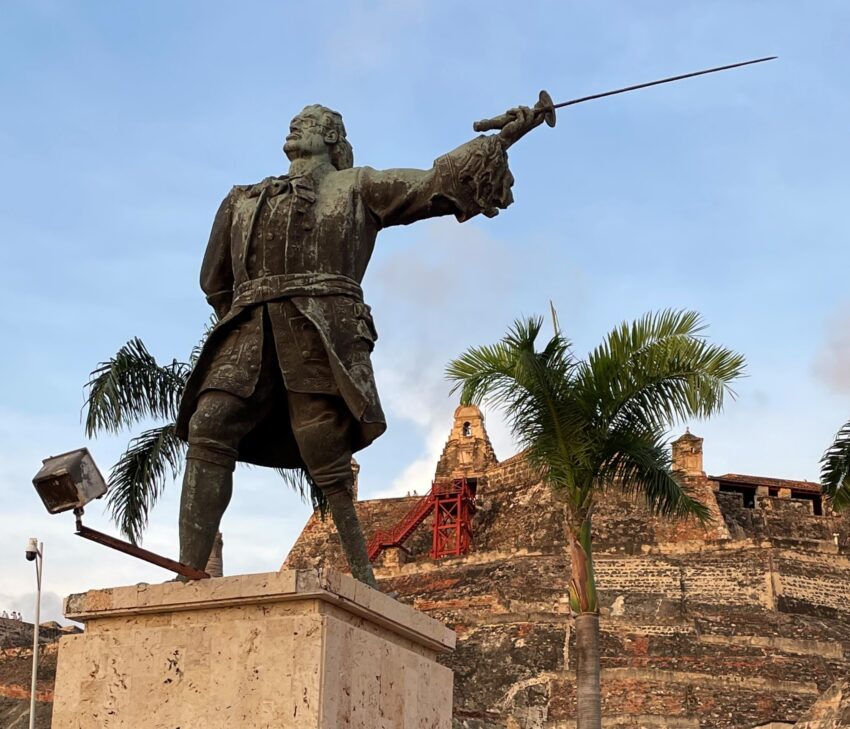The image depicts a detailed bronze statue of a man standing on a concrete pedestal with a floodlight intended for nighttime illumination positioned at its base. The statue, aged to a greenish-black patina, features the man clad in vintage 16th-century attire—a large overcoat with a sash around his waist, high boots, and a peg leg. He has long hair and his right hand rests on his hip or behind his back while his left hand proudly brandishes a thin, rapier-like sword. The background showcases a clear blue sky dotted with a few wispy gray and white clouds. Surrounding the statue, there are several palm trees and the partially visible structure of an ancient, deteriorating fortress, likely undergoing restoration efforts evidenced by nearby construction elements. The serene outdoor scene is picturesque, blending historical intrigue with natural beauty.